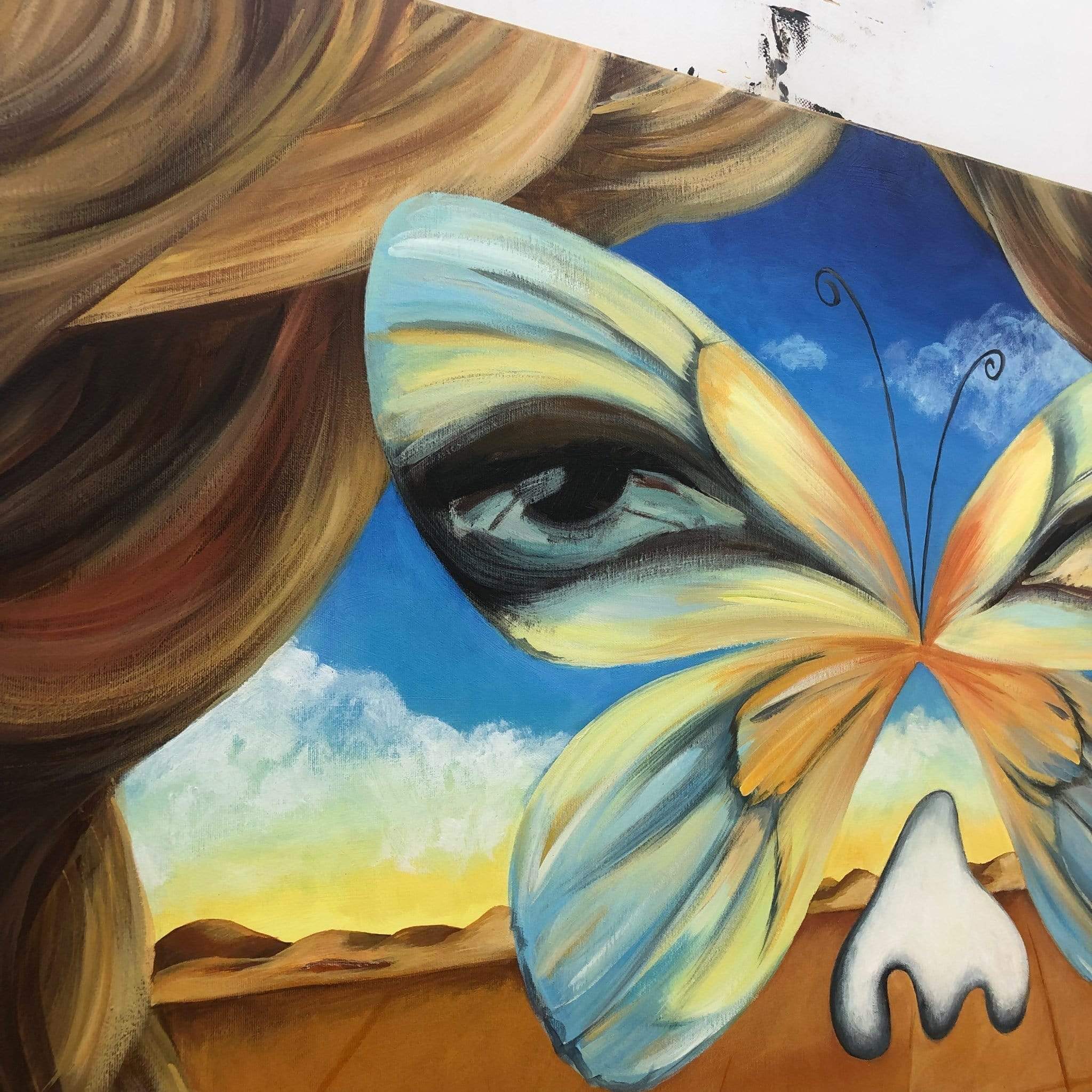The image presents an abstract painting featuring a vivid and surreal composition. Dominating the right side of the vertical rectangular canvas is a large, intricately detailed butterfly with wings in shades of orange, yellow, and blue. Notably, the butterfly's wings incorporate a realistic depiction of a human eye, complete with a dark gray and black iris surrounded by blue, adding an eerie, lifelike quality. The butterfly has two antennae; the left one is longer and curls up and around, creating a dynamic sense of movement.

Flowing from the upper left-hand corner and cascading downwards are waves of brown shades, resembling wavy, human-like hair or fabric, adding texture and depth to the painting. These waves appear almost three-dimensional, contributing to the illusion of a woman's face taking shape from the artistic elements combined within the image.

The background transitions from brown hills and desert-like land at the bottom, blending into a blue sky with white clouds suspended above, further enhancing the dreamlike quality. The painting is devoid of text, focusing purely on the visual interplay of natural and human elements to form a harmonious, yet mystifying, scene.